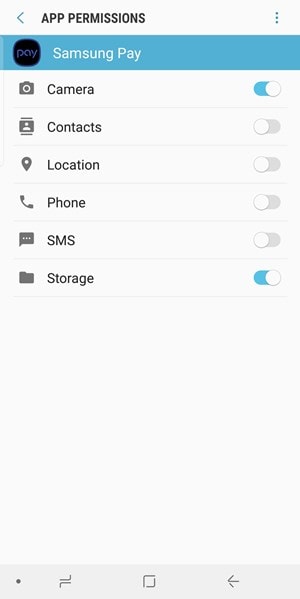The image displays a smartphone screen showcasing the app permissions settings for the Samsung Pay application. The background of the screen is predominantly white, with the header featuring the text "App permissions" at the top. Below the header, there is a section with a blue background that includes the Samsung Pay logo, which is designed in black with a purple "P" embedded in the icon.

The permissions options listed include: Camera, Contacts, Location, Phone, SMS, and Storage. The Camera and Storage permissions are enabled, indicated by the blue toggle switches positioned to the right. The other permissions (Contacts, Location, Phone, and SMS) are disabled, as their toggle switches are grey and positioned to the left.

At the bottom of the screen, there are grey-colored icons for the smartphone's navigation buttons: Home, Recent Apps, and Back. Additionally, on the top right corner of the screen, a blue icon with three vertical dots represents the options button, while the top left corner contains a back button. The overall background is a light grey, providing a subtle contrast to the elements on the screen.